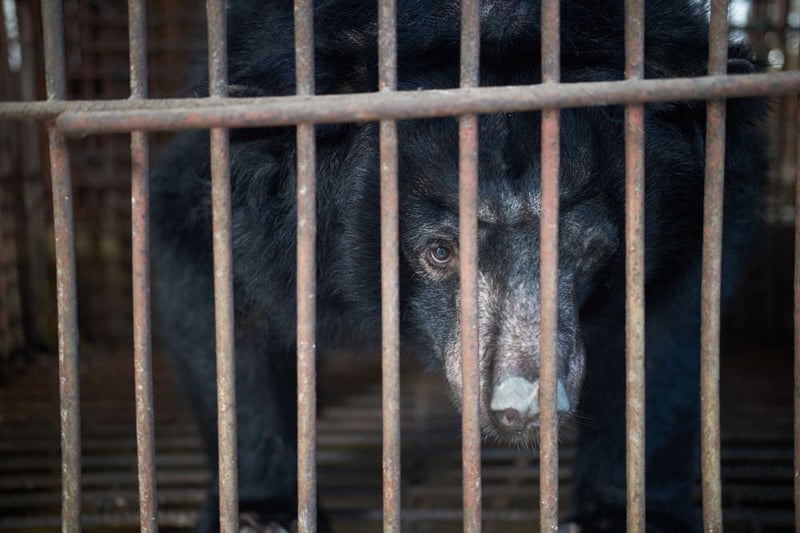The image showcases a close-up of a small black bear confined within a rusty metal cage. The bear, standing on all fours, directs its gaze straight at the camera with a somber expression. Its black, wiry fur transitions to a pale, almost milky white around the top of its nose. The photograph captures the bear peering through thin, vertical metal bars, which display significant rust. There are approximately nine to ten vertical bars and one horizontal bar intersecting in front of the bear. The background remains indistinct due to the close-up nature of the shot, only revealing additional metal bars of the same style, and possibly some daylight filtering through, suggesting the image was taken during the day. The setting could likely be a zoo or a shelter, though the specifics are unclear. The visible eye of the bear hints it may be missing the other, or it could be an issue of the angle from which the photograph was taken.